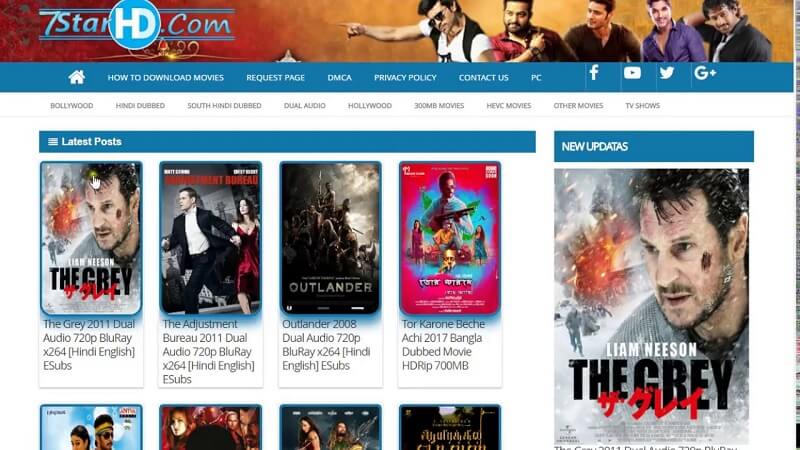This detailed caption targets what the image features and contextualizes its elements better:

---

The screenshot appears to be from a website called 7starhd.com, which is likely an illegal movie download site. 

At the top, there is a gradient bar transitioning from black on the left to a lighter red and then orange on the right. On the far right of this bar, there are five men of Indian descent dressed in various colors: the first in white, the second in black, the third in black, the fourth in blue, and the last one in black again.

The website's logo "7starhd.com" is displayed in blue text, with "HD" enclosed in a blue circle and written in white. Below the logo, there's a navigation menu featuring a white and blue bar with white text, listing options such as "How to Download Movies," "Patrocrats," "DMCA," "Privacy Policy," "Contact Us," and "PC." Also visible are icons linking to social media platforms like Facebook Global, YouTube, Twitter, and Google Plus.

The main content area has a white background with blue text that lists categories such as Bollywood, Hindi Dubbed, South Hindi Dubbed, Dual Audio, Hollywood, 300MB Movies, HEVC Movies, Other Movies, and TV Shows. There is a section titled "Latest Posts," marked by three lines, and a similar section on the right labeled "New Datas."

The image also displays thumbnails of films available for download. Prominently featured is a poster for "The Grey" (2011), depicting Liam Neeson bruised and fighting wolves. Below this, it reads "The Grey, 2011, Dual Audio, 720p, Blu-ray, X236, Hindi English." Other visible movie titles include "The Adjustment Bureau," "Outlander," "Torakani Beach," and several other unreadable titles.